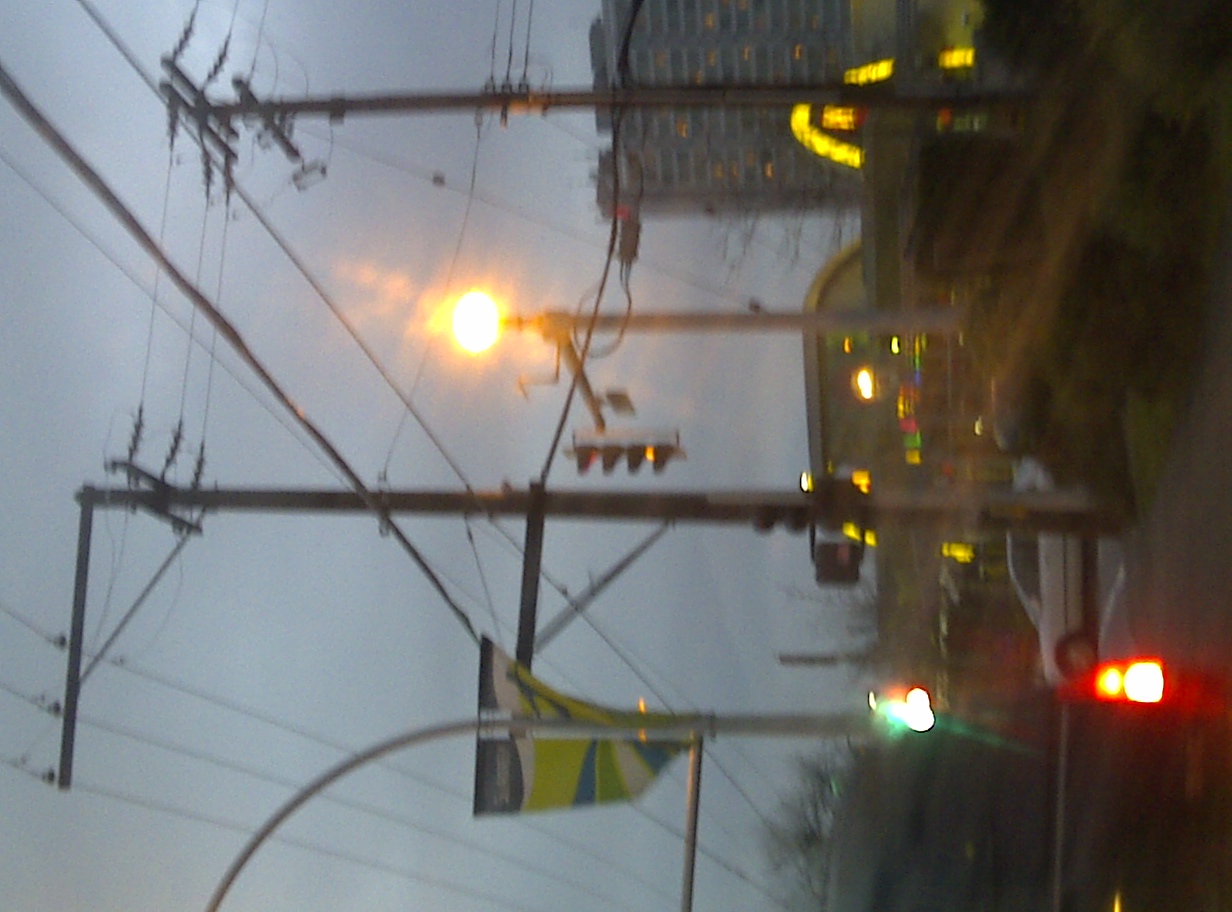A nighttime photograph captures a cityscape at dusk, bathed in a hazy blue-gray hue. The upper section of the image showcases a grouping of four upright utility poles, two of which bear the majority of the intersecting wires, contributing to the urban tapestry. Among these poles is a lighter gray one topped with a globe light, emitting a warm, golden-yellow glow that diffuses gently into the atmosphere, tinged with a peachy undertone.

Extending from this pole to the left is an arm holding a traffic light with four openings, the bottom one shining a light yellow. Below this, the cityscape unfolds in soft focus, either due to pollution or the natural haze of dusk. On the right-hand side of the frame, the iconic yellow arches of a McDonald's can be seen, juxtaposed against a tall, gray high-rise, its windows warmly lit from within. In the foreground, a white car is noticeable, accompanied by a gray pickup truck to its left, its red taillight emitting a stark contrast against the subdued tones of the evening scene.